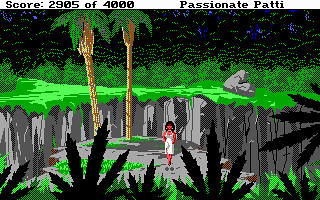This is a screenshot from a 16-bit style video game, reminiscent of old gaming systems like the Game Boy. The scene is framed horizontally with a white bar at the top displaying "Score: 2905 of 4000" and the title "Passionate Patty". The foreground is dominated by the black silhouettes of jagged plants with large and short leaves, transitioning to dark green and then light green foliage. In the center stands a woman with reddish-pink skin, short black hair, and small turquoise earrings. She wears a form-fitting white dress that cuts at the knee and has her left arm extended while the right arm is behind her back, facing the viewer. The backdrop features two large, light brown palm trees with dark green fronds, set against a cliff that alternates between light and dark gray. Atop the cliff, patches of light and dark green grass mix with a line of predominantly dark green bushes interspersed with lighter greens for depth. There’s a large grey boulder to the right and additional tree lines in dark blue or black, dotted with light green highlights indicating depth. Small purple dots are visible on both sides of the scene.